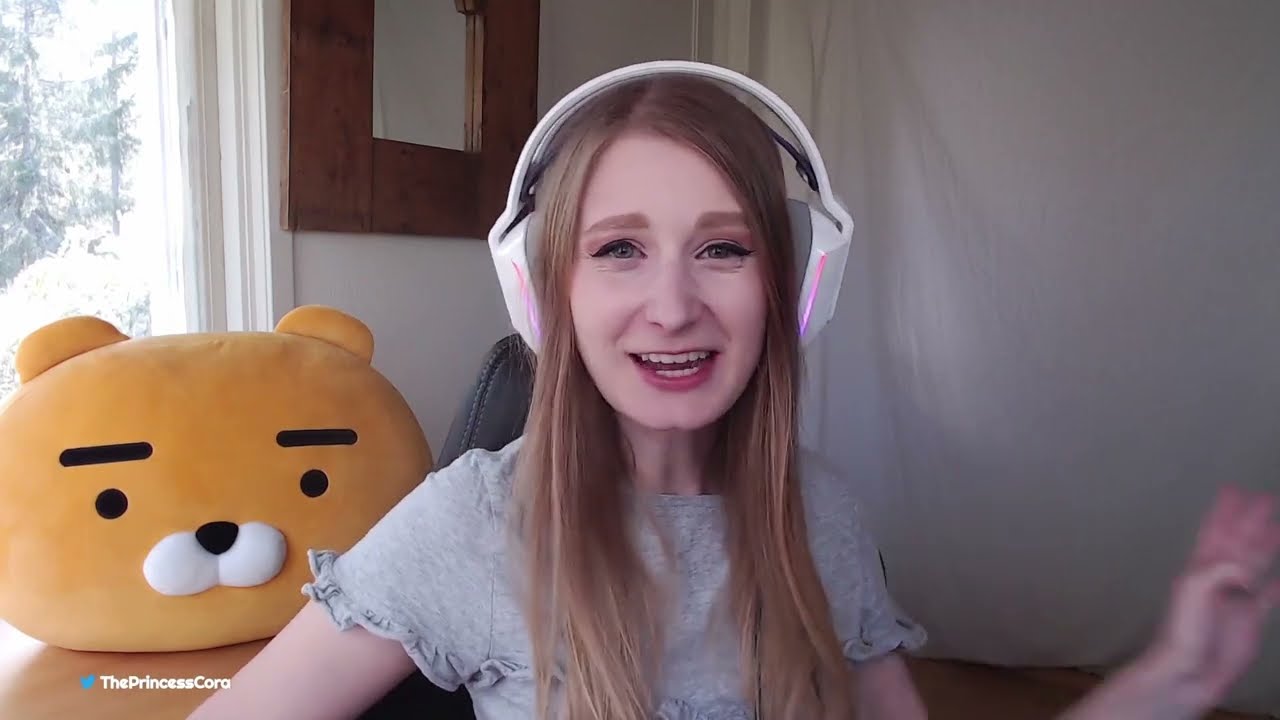A young, slender white woman with blonde hair and light complexion is prominently featured in the center of the image, facing the camera. She has light-colored eyes and is wearing sleek, futuristic white headphones with pink sidebars. She sports a light gray short-sleeved shirt. Her left hand is raised, suggesting she's moving to music. To her left on a table is a plush toy resembling Winnie the Pooh, characterized by a yellow and orange body with a neutral expression. Behind her, there's a white wall and a window that reveals a view of trees and woods outside. Additionally, to the left of the image, there's a mirror, and to the back right, a curtain. A photo frame with a thick brown border is also visible behind her. The overall hues in the image include white, brown, light golden, gray, and pink. The caption at the bottom left reads "the princess Coro."